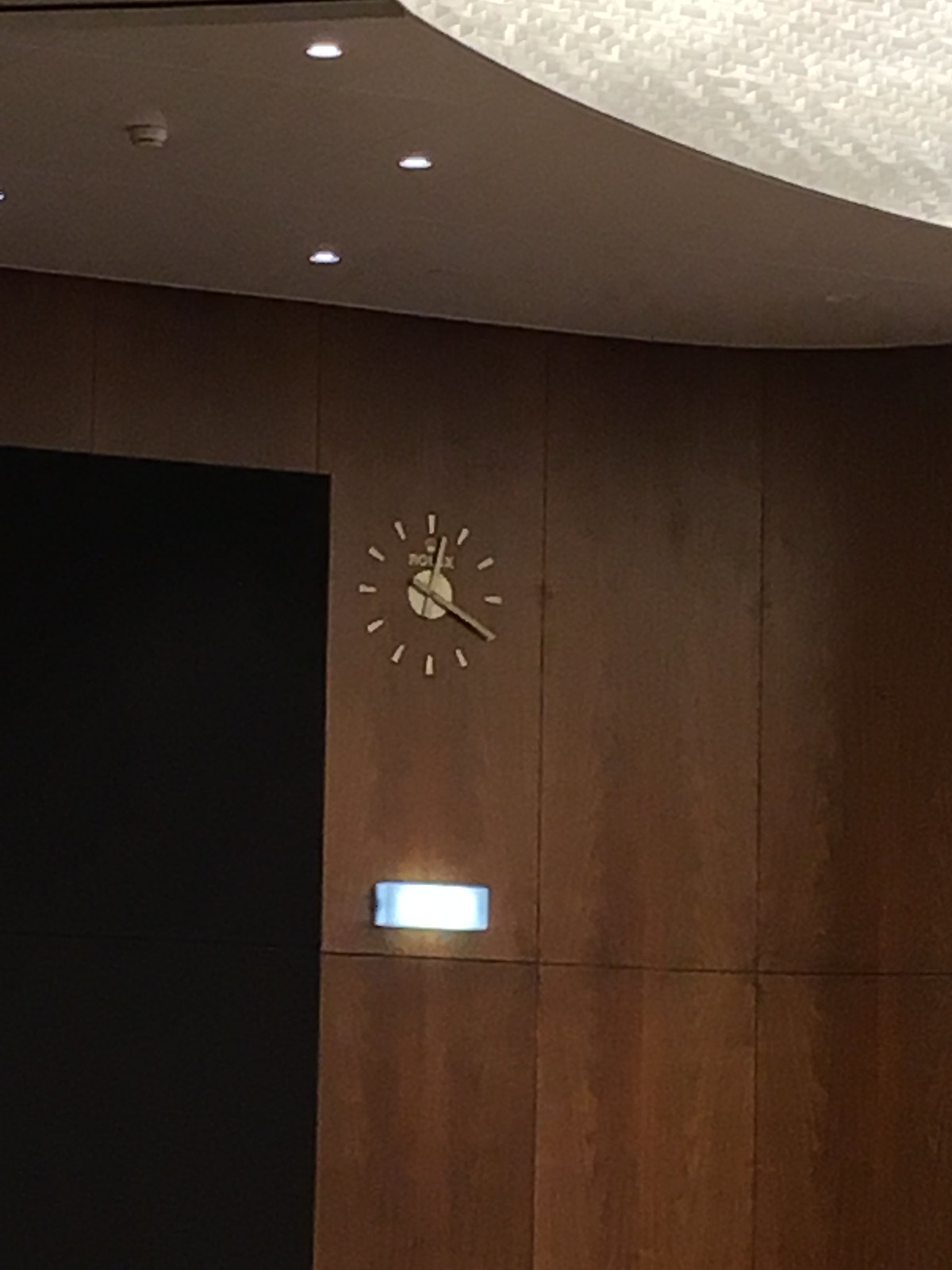This photograph showcases the interior of what appears to be a high-end building, possibly linked to the Rolex watch company. Prominent dark brown wood paneling stretches from floor to ceiling, structured in two rows of three panels each. Centered on the upper left panel is a gold or bronze-colored clock, elegantly embedded into the wood, featuring no numbers but distinct brass or gold watch hands indicating the time at 12:20. Below the clock, a waist-high light illuminates the area. To the left of the clock and light, a dark doorway suggests it might lead to an elevator. The paneled ceiling boasts three track lights and a smoke detector, adding to the sophisticated atmosphere. Above this setup, there is an additional wall leading up to a second-floor view, enriching the architectural depth of the scene.